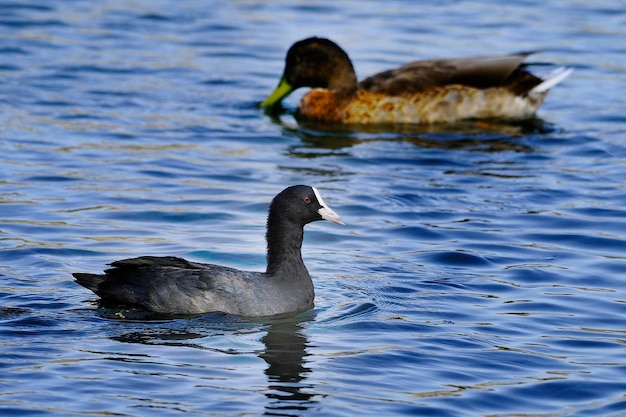In this captivating close-up image, two ducks glide on a calm and slightly rippled body of water, likely a lake. The duck in the foreground, which appears to be female, boasts dark grayish-black plumage with a distinctive white forehead and beak, and is swimming to the right. In contrast, the larger duck in the background, possibly a male, features a dark brown or black head, a brown body with a red mottled chest and belly, and a green-tipped beak partially submerged in the water as it swims to the left. The serene water captures the sunlight, reflecting the shadows of the ducks and adding a tranquil ambiance to the scene. The gentle ripples indicate a slight breeze, enhancing the natural beauty of this intimate wildlife moment.